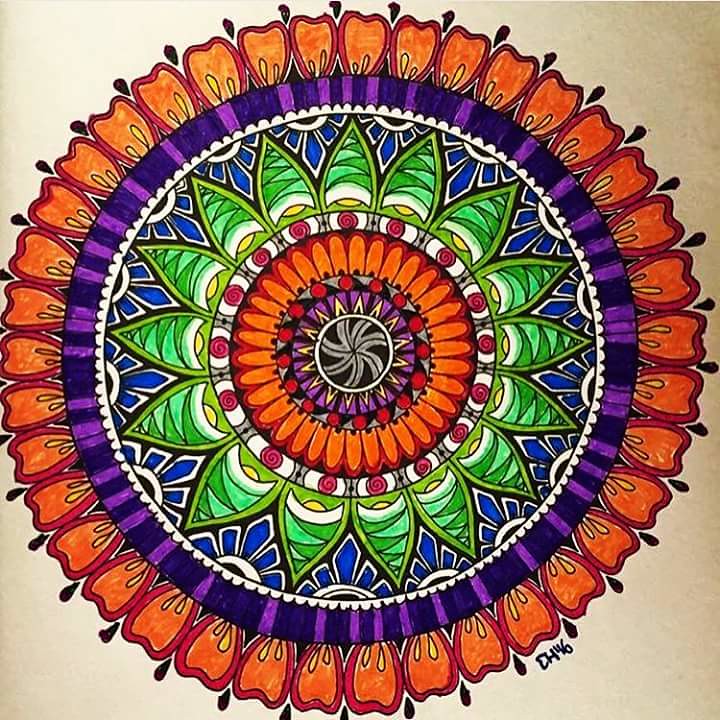In this vibrant and intricately detailed Mandala design, meticulously drawn on paper with colored markers or colored pencils, a mesmerizing array of colors and patterns come to life. At the very center lies a striking gray and black spiral pinwheel pattern, encircled by a pristine white ring. Radiating outward from this focal point are vivid yellow spikes, followed by a smooth purple ring. A series of bold red circles form the next layer, transitioning seamlessly into a line of orange and red oval shapes.

Further outward, red and white spirals create a sense of dynamic motion, from which green petals burst forth, their forms elegantly filled with delicate blue flower patterns. This visually engaging layer is encased by a purple and blue ring, adding a soothing balance to the composition. Finally, the outermost ring captivates with its resemblance to orange petals, each highlighted by red trim, completing this stunning and harmonious Mandala masterpiece.